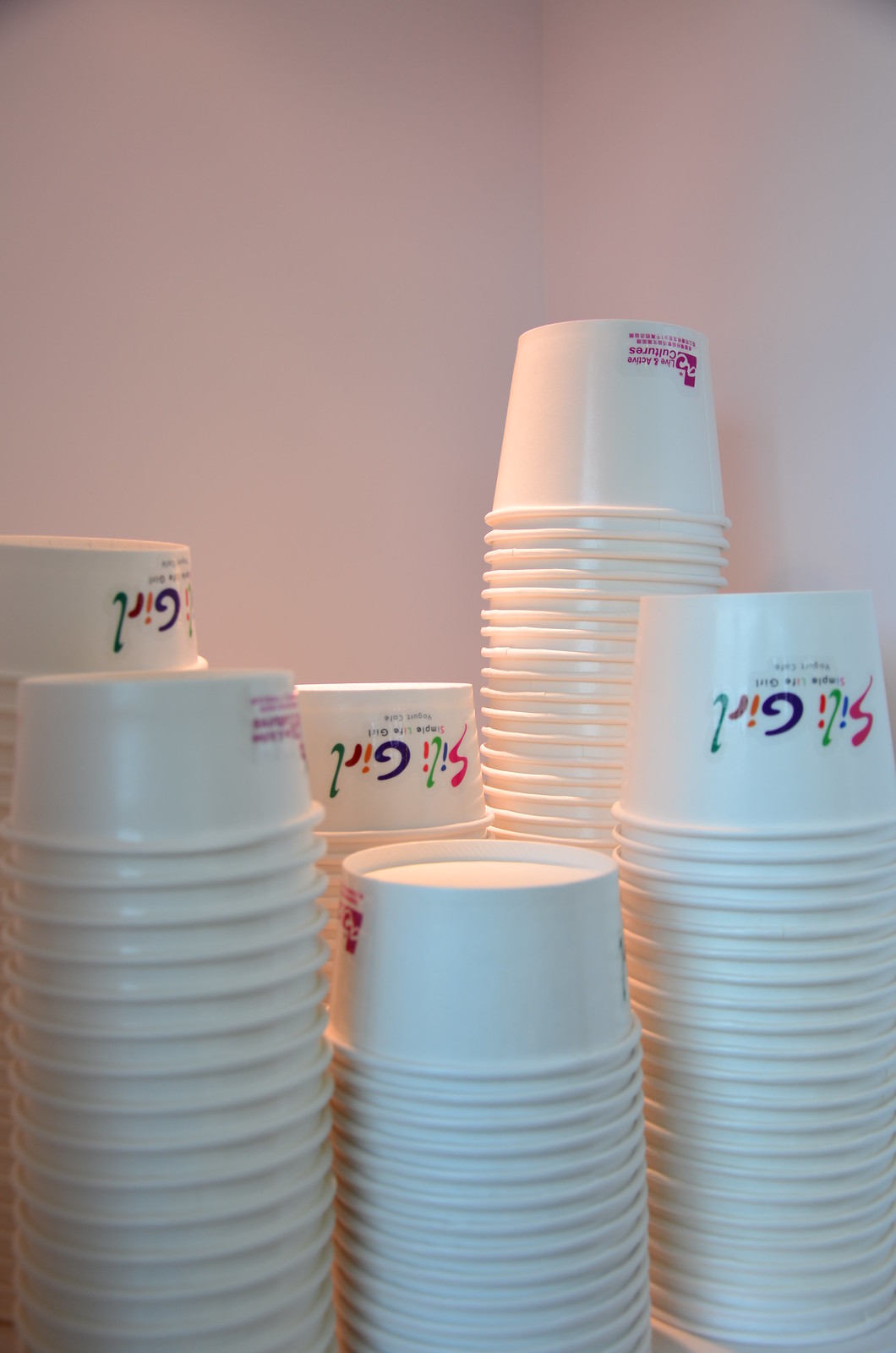This photograph features a clean, white background, possibly a corner wall, with six stacks of white cups of varying heights arranged in a neat display. The cups appear to be made from a material similar to wax or styrofoam, commonly associated with frozen yogurt or ice cream. Each cup prominently displays a colorful logo featuring the words "Silly Girl" in pink, blue, green, orange, and purple letters. Below this logo, it says "Simple Life Girl Something Cool." The cups come in three different sizes, presumably small, medium, and large, all meticulously stacked and ready for use, evoking the feel of a frozen yogurt shop.